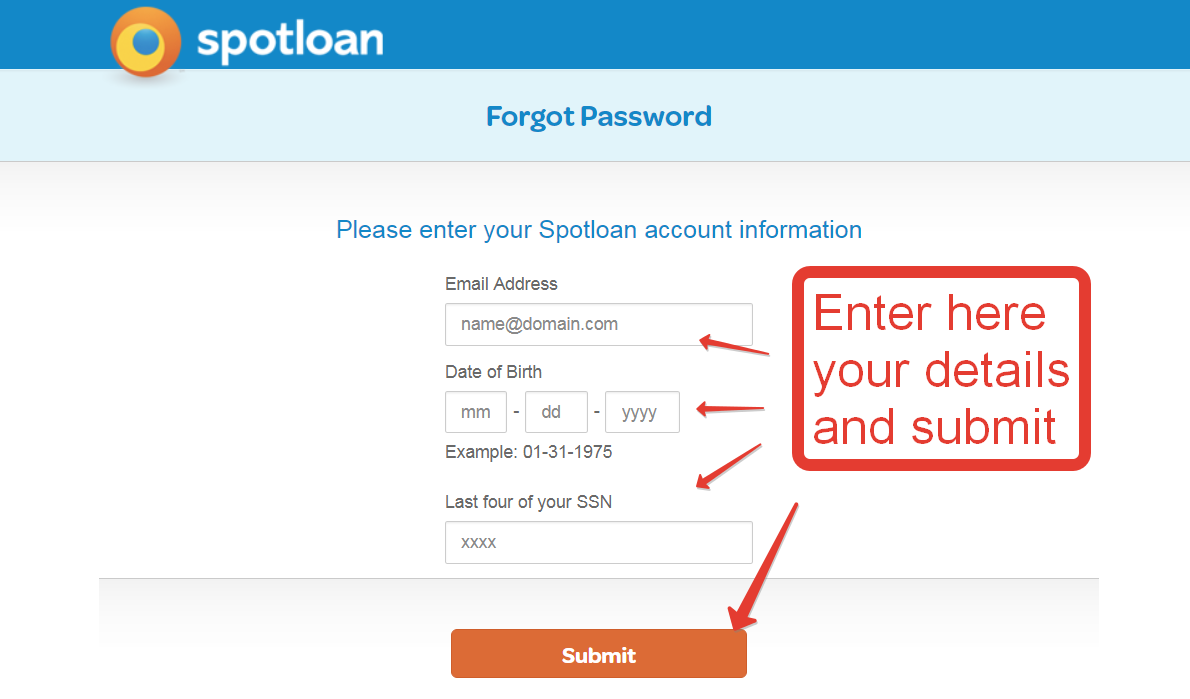The image features a web page layout with a predominantly blue-themed header. At the top left of the header, the word "Spotlone" is displayed in white text. Accompanying the "S" of "Spotlone" is a circle representing the letter "O," featuring an orange outer ring and a yellow inner fill.

Below the header, centered on the page, appears the text "Forgot Password," also in blue, set against a contrasting light blue background. Following this section is the main page content, starting with the instruction: "Please enter your Spotlone account information" written in blue.

The form consists of several input fields:
1. **Email Address**: A labeled input space prompting users to enter their email, illustrated by an example: "name@domain.com."
2. **Date of Birth**: Formatted as month, day, year, with an example: "01-31-1975."
3. **Last Four of Your SSN**: A space for the last four digits of the user's Social Security Number, illustrated with four 'X's.

At the bottom of the form is an orange "Submit" button with white text, set against a slightly gray background for enhanced visibility.

On the right side of the form, a red square contains additional information: "Enter here your details and submit." Surrounding this text, there are four red arrows that point to different parts of the form:
- One arrow directs attention to the "Email Address" field.
- Another highlights the "Date of Birth" field.
- The third arrow points to the "Enter your SSN" field.
- The final arrow guides users towards the "Submit" button at the bottom of the form.